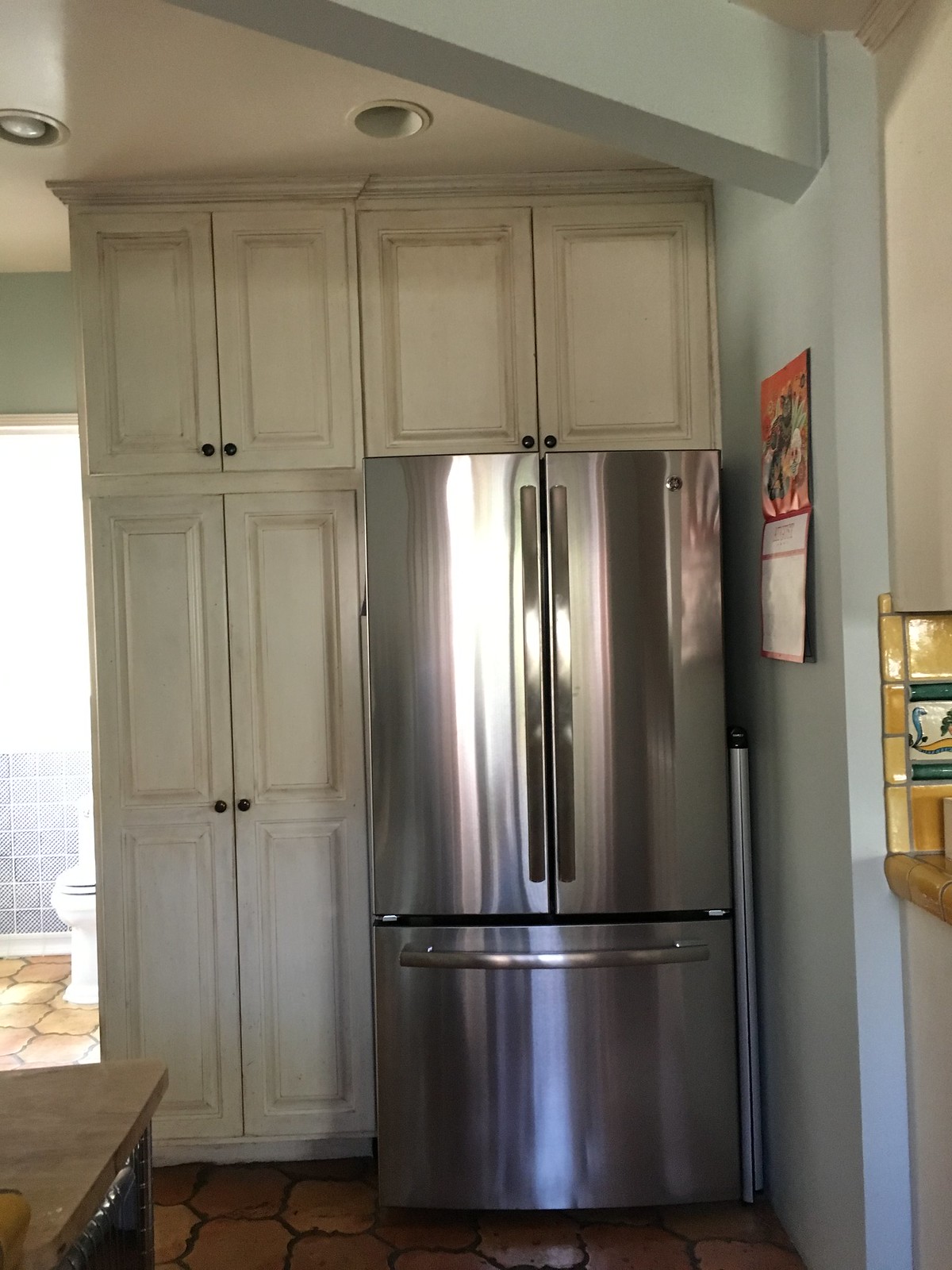The image depicts a segment of a kitchen with a light blue wall and white cabinets. Central to the image is a stainless steel refrigerator-freezer combination, with a bottom freezer that features a pull-out handle, and a side-by-side split refrigerator on top. To the left of the fridge are two sets of cabinets: a tall set almost reaching the fridge’s height and a smaller pair above it. Both sets are a beige-tan color with black knobs. Above the refrigerator, there are additional tan cabinets with black knobs. A light green wall, with a calendar displaying orange and black imagery, flanks the right side of the refrigerator. Brown and tan tiles cover the kitchen floor. In the background, light spills into the kitchen from an open doorway revealing a bathroom. The bathroom features a white toilet with a closed lid, set against blue tiled walls with white trim.